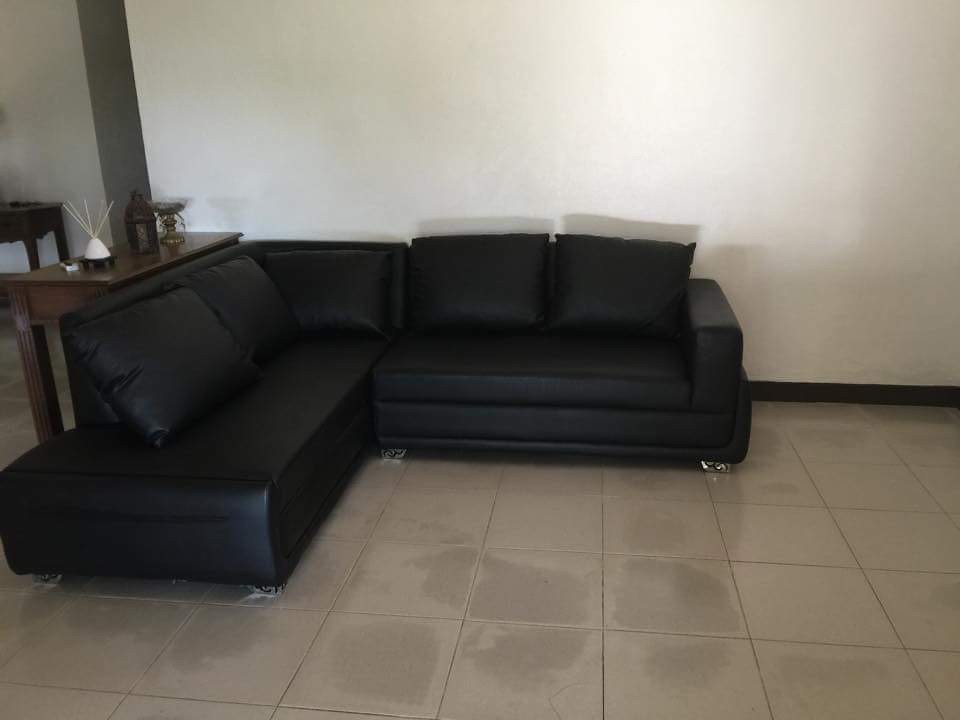The image depicts a dimly lit interior room featuring an L-shaped black sofa that is positioned at a 90-degree angle, serving as the focal point. The sofa, located closer to a light gray or white-painted wall, includes two sections—one longer on the left—along with a couple of black pillows adding to its plush appearance. In front of the sofa, the floor is covered in off-white or gray square tiles arranged in vertical rows. Adjacent to the sofa, there's a dark brown wooden end table adorned with a few small, indistinct objects or knick-knacks. Further in the background, another table is visible, adding depth to the scene. A black baseboard runs along the right-hand side of the image, complementing the overall monotone color palette. Subtle shadows on the wall reflect the arrangement of the furniture, enhancing the serene and muted ambiance of the room.